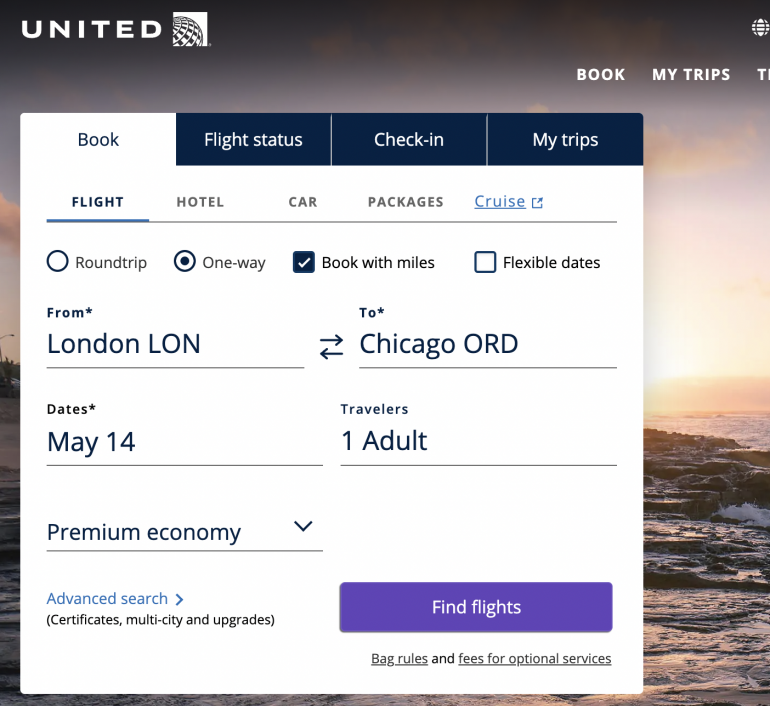On the United Airlines booking website, prominently displayed in the top left corner is the United Airlines logo. The page is partially cut off on the right side, but you can still see tabs for "Book" and "My Trips." The background features a picturesque image of a body of water at sunset. 

The selected tab is "Book," and within this section, there are options for booking flights, hotels, cars, package deals, and cruises. The "Flight" option is currently selected, displaying preferences for round-trip or one-way tickets, with one-way being chosen. Additional options include "Book with miles" and a flexible dates feature. 

The travel itinerary is set from London to Chicago on May 14th for one adult traveler. The booking class is set to premium economy. There is also a button available to initiate the search for available flights.